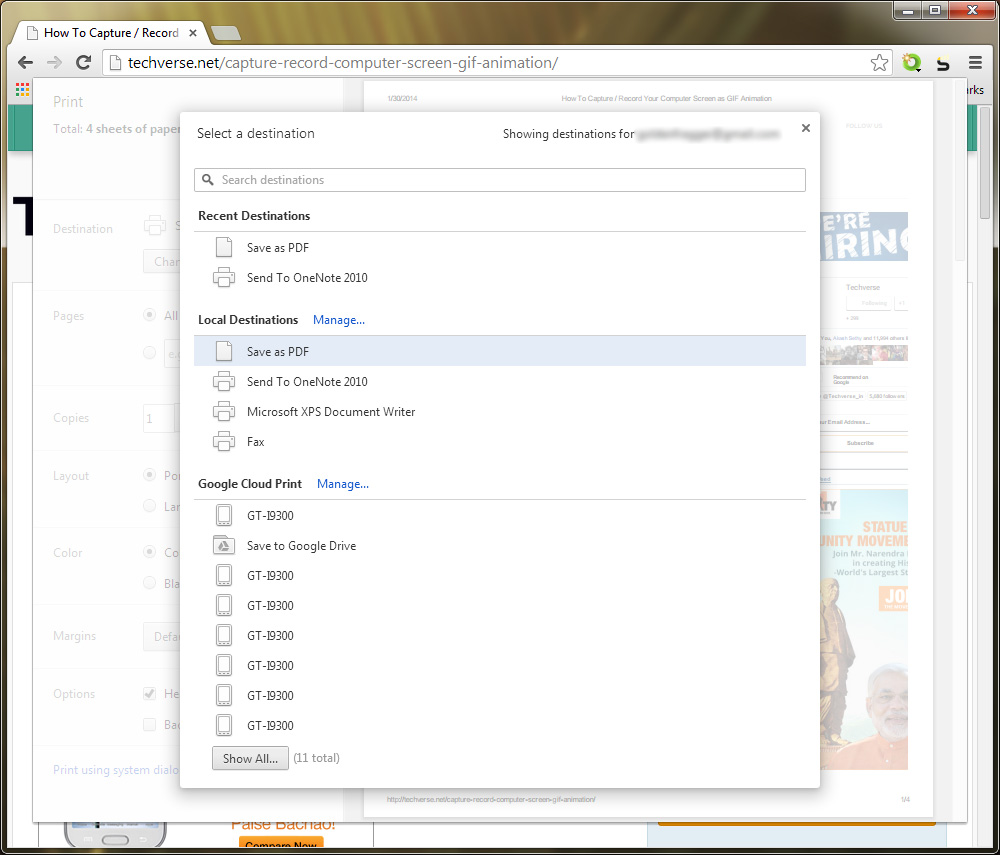This image is a cropped screenshot of a computer desktop screen, densely packed with multiple tabs. Dominating the center is a large white dialog box labeled "Selected Destination" in the top left corner. Next to it, "Showing Destinations For" is followed by pixelation to protect personal information. Below this header is a prominent search bar labeled "Search Destinations."

The layout continues with a bold section titled "Recent Destinations," listing two options beneath it. Further down, the "Local Destinations" section, also in bold, features a "Manage" hyperlink in blue font to its right. Under this section are three or four options, with "Save as PDF" currently selected.

The third category within this dialog box is named "Google Cloud Print." It also includes a "Manage" hyperlink, with a vertical list of options below it. At the bottom left of the box, a button labeled "Show All" is accompanied by the text "(11 total)" in parentheses.

In the background, partially obscured by the dialog box, is a computer print screen window. The larger backdrop is headed by "Print" in the top left, with a print preview image to the right. The browser tab in the upper corner indicates the user is capturing or recording a computer screen GIF animation.